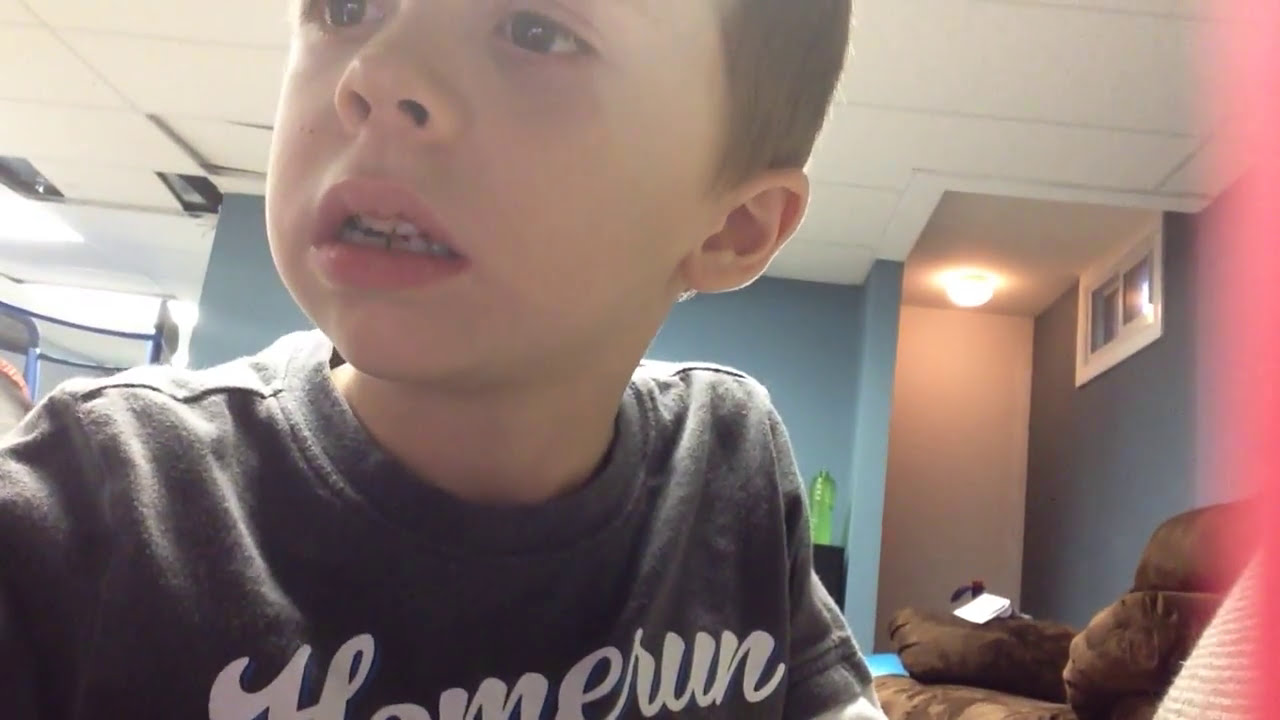A photograph depicts a young boy, likely around four to six years old, with very pale skin and short brown hair. He is wearing a dark gray t-shirt with the white cursive words "Home Run" on it. The boy's mouth is slightly open as he gazes towards something off to the left side of the image. He stands in a room with light blue painted walls and a mostly white ceiling. A pink light or object is faintly visible on the right side of the image, adding a subtle glow to the setting. Directly beside the boy, on his right, is a brown sofa or armchair with a white book resting on one of its arms. The background reveals elements of a lived-in home, including small windows, a green sports drink container, and possibly bunk beds in the distance. Additionally, there are framed artworks on the right wall, and on the left wall, a mini split air conditioner can be seen. Overall, the image captures a moment of quiet observation by the young boy in a cozy, colorful room.